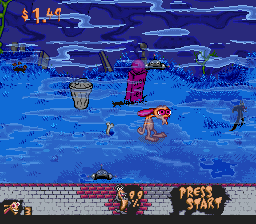This is a detailed screenshot from an older video game, likely from the early Nintendo systems. The game's graphics are reminiscent of a side-scroller with depth, creating a dark, eerie atmosphere. The screen features a character that resembles the dog from the Ren and Stimpy show, possibly Ren, trudging through a barren, desert-like environment. A variety of colors, particularly varying shades of blue, gray, purple, and red, make up the sky and the brick-like ground.

In the top left corner, there is text displaying "$1.49," suggesting in-game currency. The bottom left corner shows three icons of Ren, indicating the number of lives left. The game interface includes a instruction to "Press Start" in light orange letters with a darker border situated in the bottom right corner. Above this, the number "99%" adds another layer of mystery to the game’s objectives, possibly indicating progress or a certain condition met. Overall, the scene suggests Ren walking under an ominous alien device, enhancing the creepy, desolate environment.